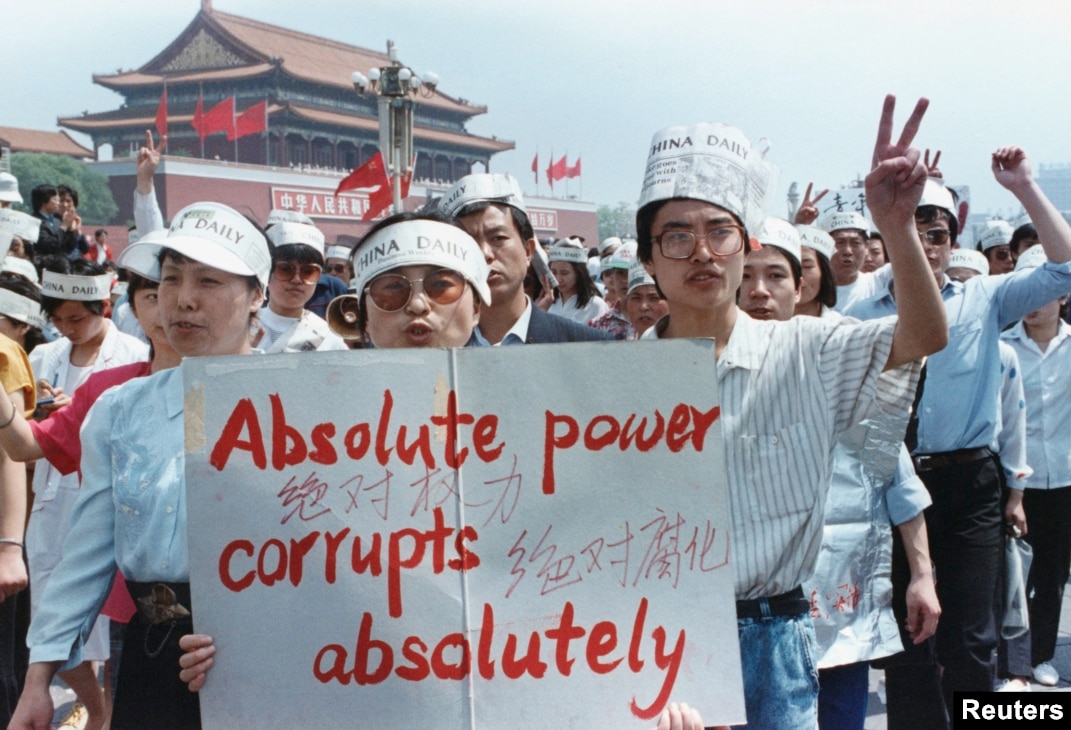This photograph captures a large protest in China, depicting a diverse group of both young men and women marching in solidarity. Prominently in the foreground, three individuals wearing hats emblazoned with "China Daily" hold up a white sign with bold orange text stating, "Absolute power corrupts absolutely," accompanied by a Chinese translation underneath. The atmosphere is charged, with participants raising fists and making peace signs, symbolizing their call for change. The lower right corner of the image bears a Reuters watermark, indicating the credibility of the source. In the background, an elegant, traditional Chinese building with a pagoda roof rises majestically, contrasting with the modern-day scene of civil unrest. Red flags wave nearby, and the sky overhead is a serene mix of light blue and white, bringing a striking contrast to the intensity of the protest below.